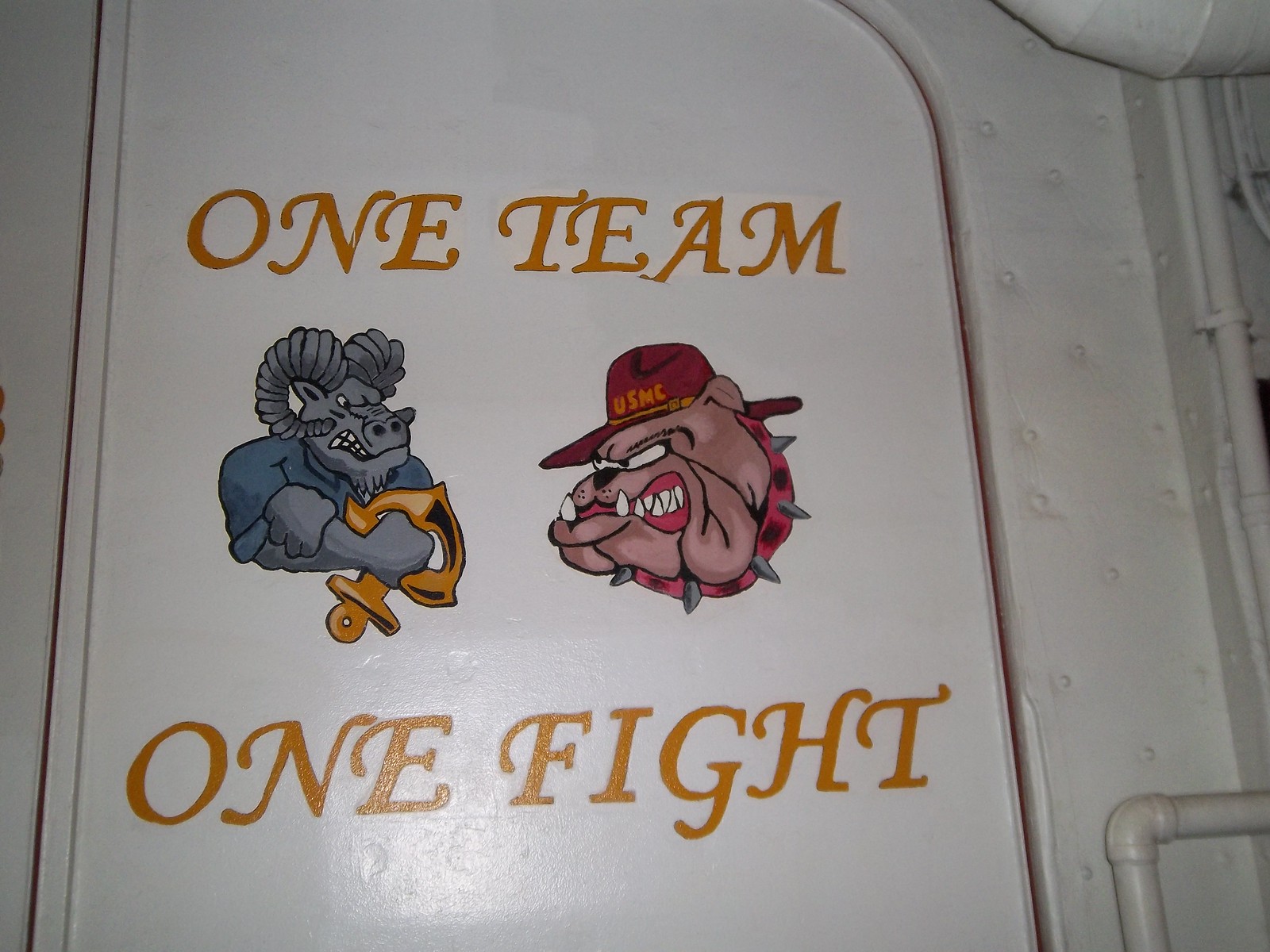This horizontal rectangular image captures a white wall accentuated by a delineated rectangular panel with rounded corners at its center. Dominating this panel, gilded text reads "One Team" above "One Fight." Between these phrases, two cartoon-style logos are featured. To the left, a gray ram, dressed in a blue shirt and holding the hilt of a sword with its blade missing, adds a dynamic element. To the right, an English bulldog sporting a spiked collar and a hat emblazoned with "USMC" in yellow, intensifies the visual narrative. The image is set indoors, possibly within a college or institutional setting. Additional elements include steel pipes or tubing visible in the upper right and lower right corners, also painted white, suggesting an industrial or utility space, perhaps a boiler room. This detailed composition melds text and imagery to convey a unified message and symbolic rivalry between two teams.